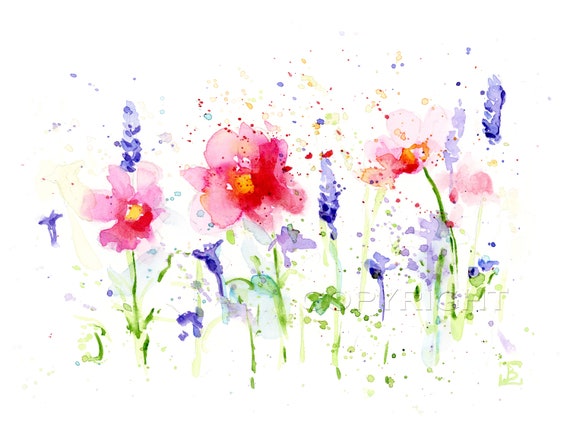This is a simple yet lively watercolor painting on a white paper background, featuring a bouquet of diverse flowers. The composition prominently displays three large pink flowers, possibly dahlias or impatiens, each with darker pink centers transitioning to yellow pistils. Interspersed among them are smaller, delicate purple flowers resembling muscari or mascarati, painted with soft, loose strokes. The green stems are depicted with fluid brushstrokes that convey a sense of natural movement. Adding a whimsical touch, the painting is adorned with multicolored paint splatters that give an impression of moisture and spontaneity. The overall effect is one of vibrant simplicity, capturing the essence of the watercolor medium. In the bottom right corner, a watermarked logo subtly blends into the scene.